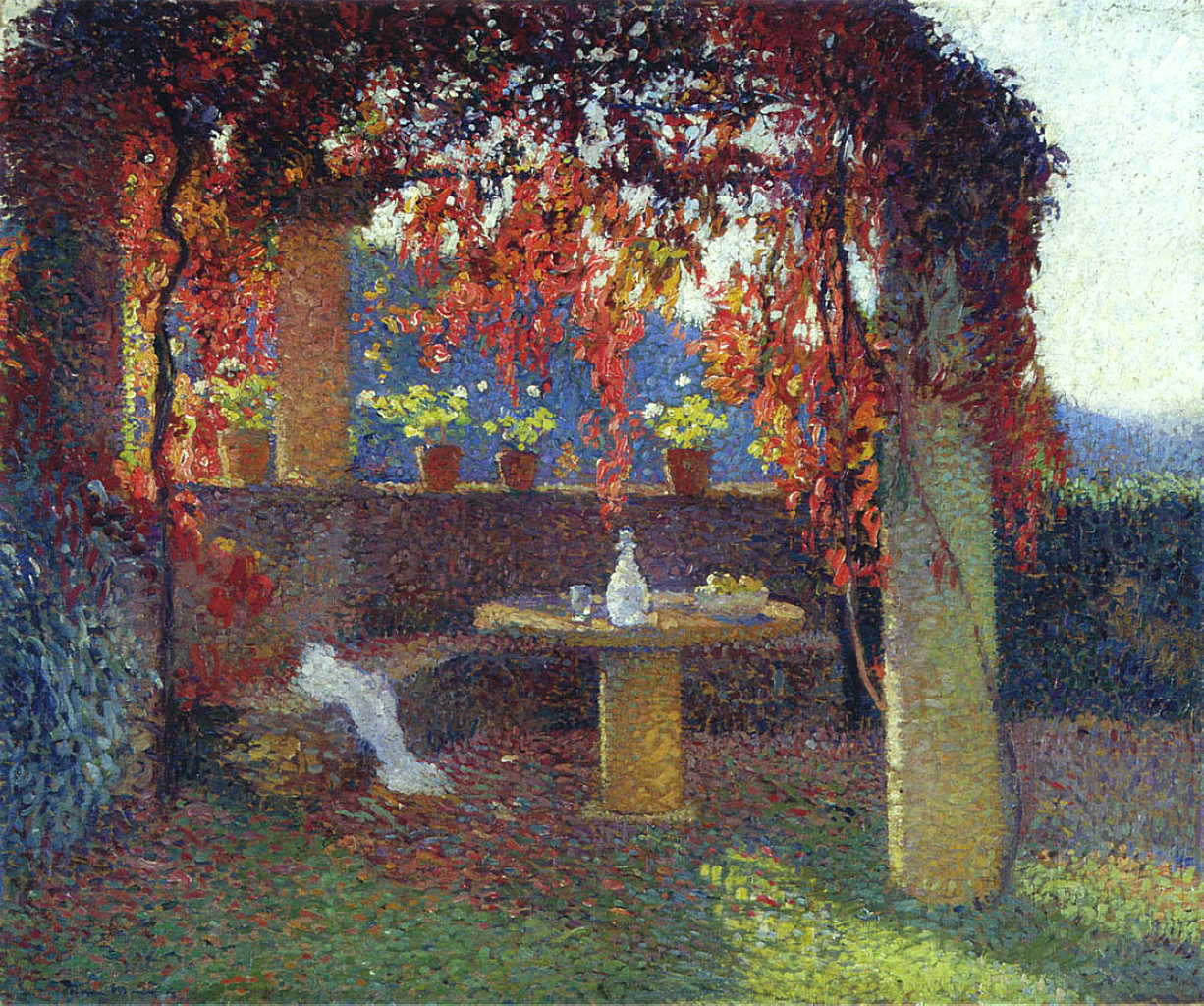This image depicts a vibrant, pointillist painting of a serene garden scene bathed in sunlight. The centerpiece is a circular wooden table adorned with a white jug, a cup, a bowl of green fruit, and some plates, all set for a garden meal. The table is located underneath a pergola or covered area supported by four pillars. This structure is beautifully draped with vines bearing red, golden, and orange leaves, reflecting the autumn season. The garden floor transitions from a grassy green outside the pergola to a reddish hue underneath it, suggestive of dappled light filtering through the foliage above. 

Flanking the table are wooden benches, one of which has a piece of white fabric draped over it. A stone wall defines the perimeter of the garden, lined with brown clay pots filled with green plants topped with white flowers. The scene is backed by a hillside under a dynamic sky showcasing shades of blue and gray. Shadows cast by the pergola add depth and realism to the painting, grounding the idyllic scene in a palpable sense of place.